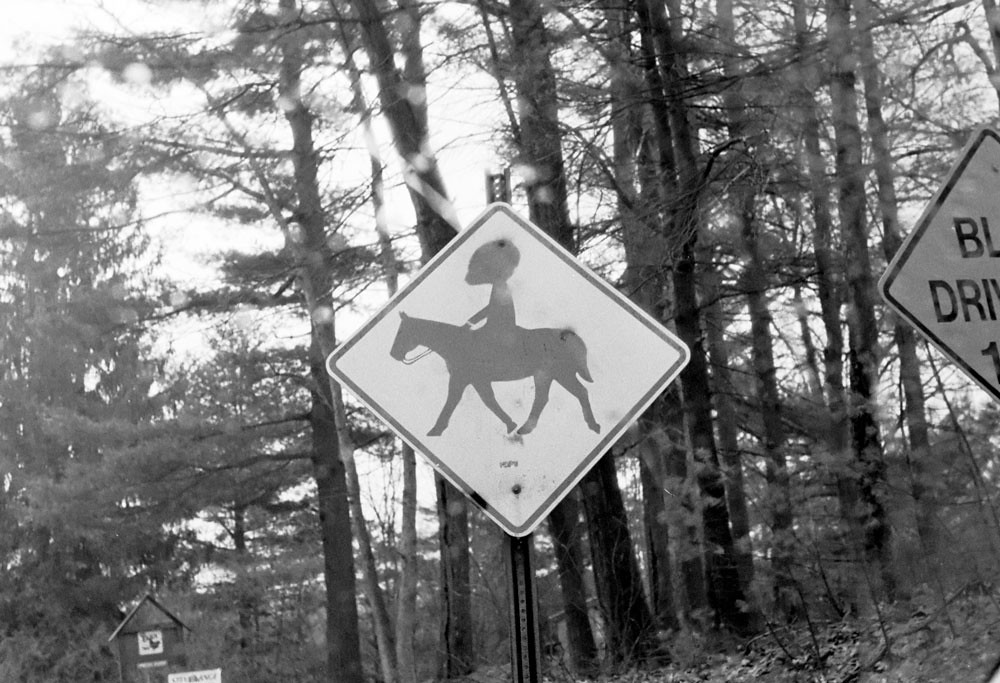In this black-and-white photograph, we are transported into a woodsy forest area lush with tall trees, some sparse in leaves while others are dense in foliage. Dominating the center of the image is a diamond-shaped sign with a black border, prominently displaying the image of a horse being ridden by a person whose head appears disproportionately large compared to their body. To the right of this, another diamond-shaped sign is only partially visible, showing the letters "BL" at the top and "DRI" below, with the rest cut off. The scene is framed by a cloudy gray sky and additional indistinct signs are visible in the background. To the left of the horseback sign, there stands a wooden structure shaped like a house with a pointed roof, topped by an unreadable white sign. The photograph skillfully captures the contrasting textures and tones of the trees, signs, and sky, creating a richly detailed scene.